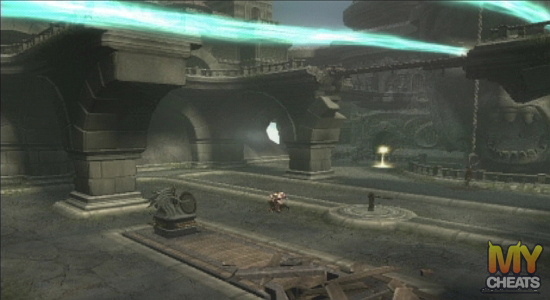The image portrays a striking scene from a video game, enveloped in a dreary, monochromatic palette with varying shades of gray. It features an ancient, somewhat ruinous architectural setting dominated by towering stone pillars, stout columns, and gracefully arched stone passageways. The ground is entirely flat, providing a stark contrast to the surrounding structures. At the center of this flat expanse stands a diminutive figure, easily overlooked amidst the grandeur of the surroundings. A notable point of interest is situated in the upper right corner, where ethereal blue lights emanate from an indistinguishable source, casting a mystic glow across the otherwise somber environment. The sky in the background is partially visible through a large aperture, suggesting an open-air or partially collapsed construction. Adjacent to this gap, a prominent white streak extends downward, cascading to meet the floor, adding a curious element to the scene’s intricate composition.